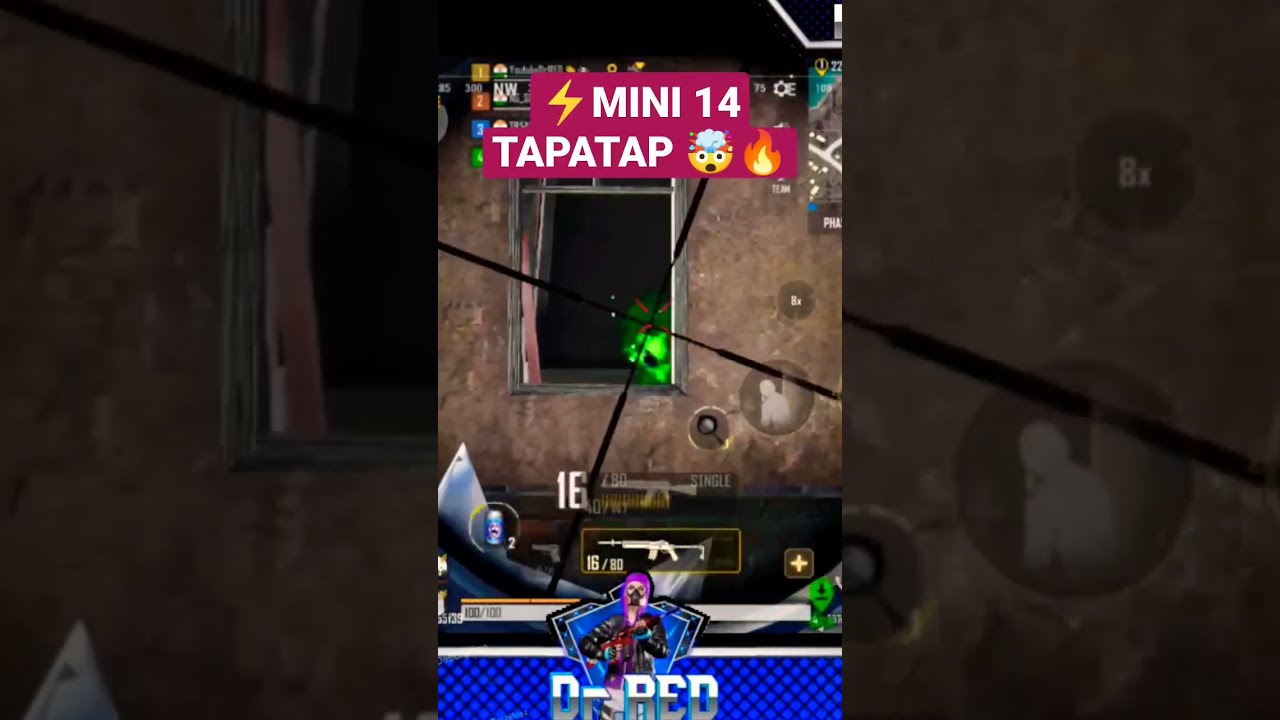The center of the image is a vertical screenshot from a video game, displayed within a stylized frame featuring semi-transparent dark borders on either side that subtly reveal the scene behind them. The screenshot captures a grungy section of a building wall with a broken wooden frame around a window. The interior of the window is pitch black, faintly illuminated by a glowing green object in its bottom right corner. Some black cables extend into the window, creating an impression of a rotated crosshair. At the bottom is a character named Dr. Red, holding a Mini14 machine gun, noted by the visible icon showcasing the gun and ammunition count of "16 out of 80". Dr. Red is depicted as an avatar with purple hair, wearing a gas mask and a black leather jacket. At the top of the screenshot, red text reads "MINI14 TAP TAP" accompanied by emojis – a concerned expression, a flame, and a mind-blowing surprise face. The details, though somewhat blurred, suggest a tense and immersive in-game scenario centered around the usage of the Mini14 weapon.